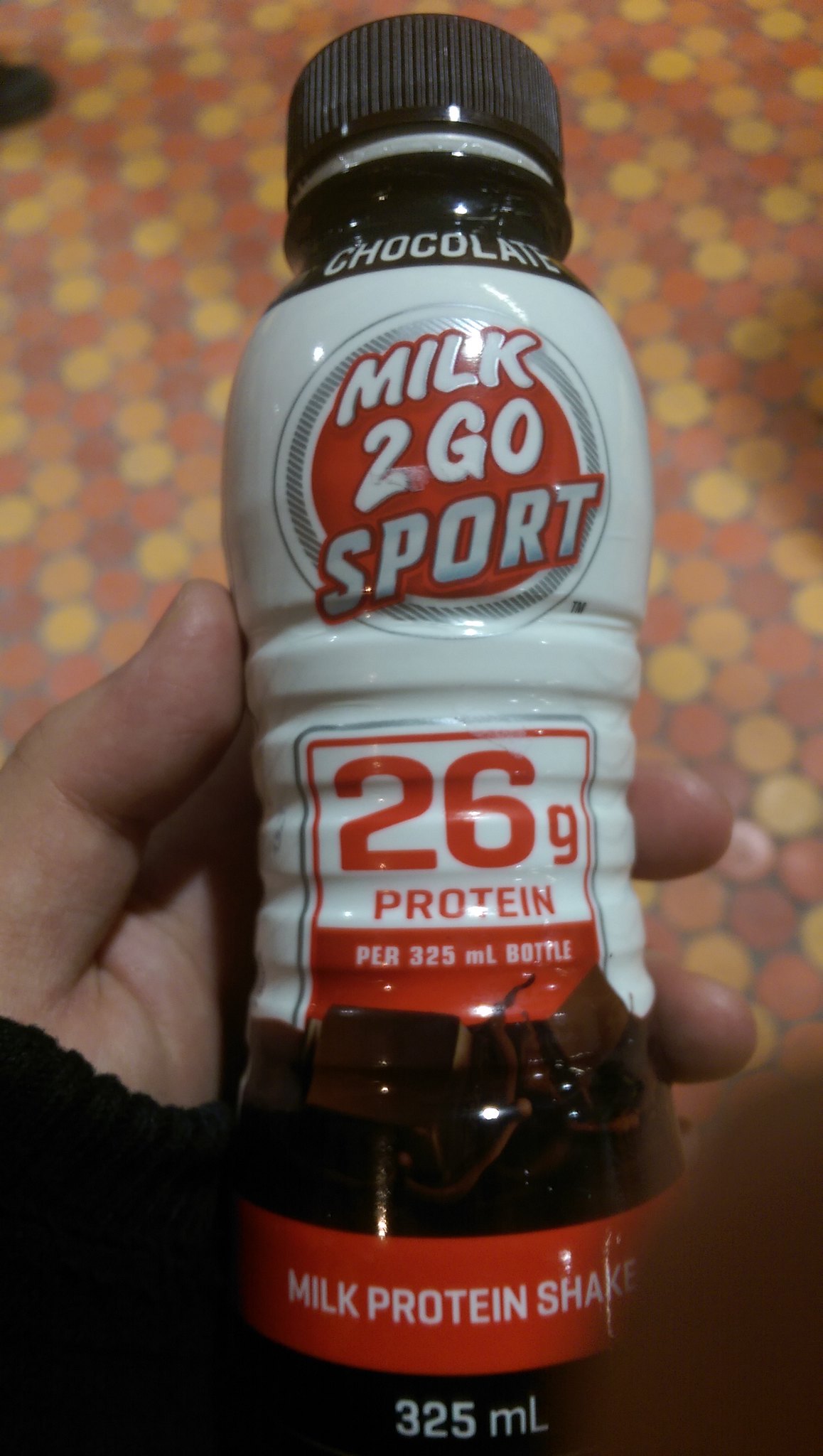The image is a close-up photograph of a packaged retail bottle of "Milk to Go Sport" chocolate-flavored milk protein shake. The bottle, which is held in someone's hand, has a black screw-top cap. The label features red and white text on a reddish circular background, prominently displaying "Milk to Go Sport" and "26 grams of protein per 325 milliliter bottle" in bold red letters. Above these, near the lid, is a black area with the word "chocolate." Below, there is a small red and white box emphasizing the protein content, along with images of chocolate bricks. The bottom portion of the label has a red strip that reads "milk protein shake" and lists the bottle's volume as 325 milliliters. The individual holding the bottle appears to be wearing a black long-sleeve sweater, and the background features a multi-colored floor with polka dots or hexagonal tiles in shades of yellow, orange, and red.